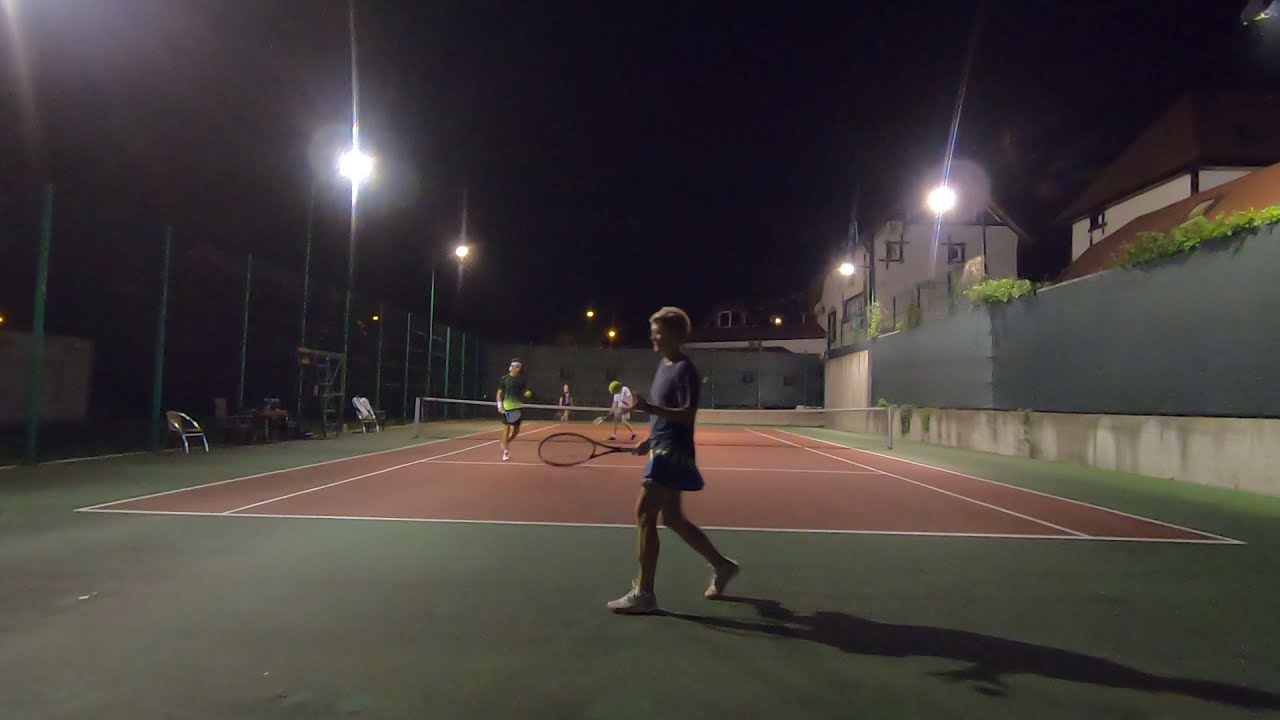The image depicts a nighttime doubles match on a recreational tennis court illuminated by several overhead lights. The sky above is pitch black, providing a stark contrast to the brightly lit court. The outer edge of the tennis court is green, while the inner playing areas are tan-colored, all marked with distinct white lines delineating the zones of play. The court is surrounded by a combination of a tall green fence on the left and chain-link fences covered with gray canvas on the back and right. To the right of the court, behind the fence, are multi-level white and brown buildings.

Within the court, four players are poised in the midst of a tennis game. The player closest to the camera is dressed in white shoes, blue shorts, and a blue short-sleeved shirt, indicating active movement towards the left side of the shot, holding a racket in his right hand and a ball in his left. Another player nearer to this primary individual wears a black shirt with a yellow bottom and gray shorts. The net spans the middle of the court, beyond which the two opposing players stand ready, one in a white shirt and the other farther back in a black shirt. Beside the court, there are a couple of chairs, hinting at a break or rest area for players or spectators. The setting hints at a possible country club environment, where facilities might include equipment rentals and refreshments.